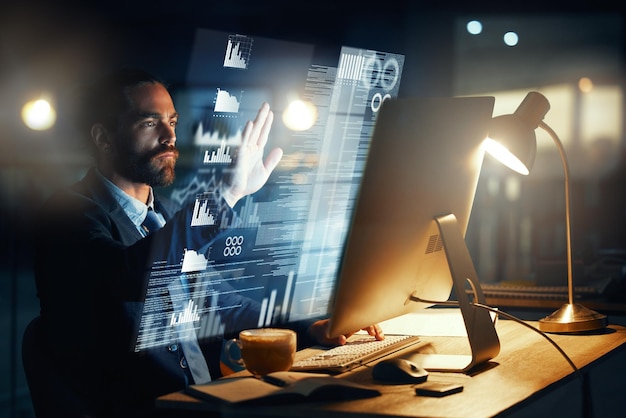In this photograph, we see a man dressed in a black suit sitting at a light wood-colored desk within a dimly lit room. The primary sources of light are a desk lamp to his right and another possible light source behind him, casting a soft, amber glow. The man is viewed from a diagonal side angle, focusing on his intense gaze directed at a 3D holographic projection emerging from a computer monitor situated in front of him. His right hand, which appears to be gloved, reaches out to interact with the vivid blue projection. The desk is organized with a keyboard, an open book, papers on the upper right, and a cup on the left. The background behind him is blurred, accentuating the man's interaction with the floating screen.